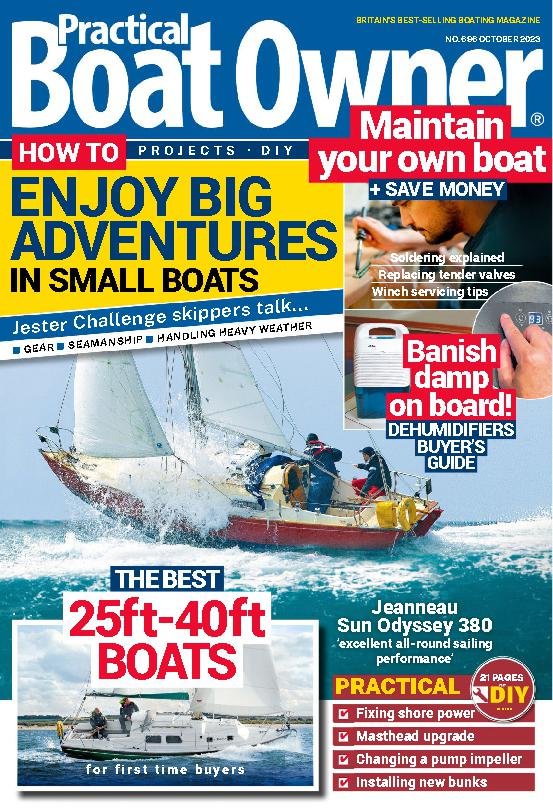The October 2023 issue of Practical Boat Owner, Britain's best-selling boating magazine, features a vibrant cover with various overlaid images and text. The top of the cover proudly displays the magazine's name in large white text, with a bold declaration of its popularity in the upper right-hand corner. The main headline encourages readers to "Enjoy Big Adventures in Small Boats," with insights from challenge skippers on gear, seamanship, and handling heavy weather. To the left, set against a yellow background, a prominent headline reads, "Maintain Your Own Boat and Save Money," highlighting articles on soldering, replacing tender valves, and winch servicing tips. Adjacent to this is an article titled "Banish Damp Onboard," offering a dehumidifiers buyer's guide. The cover also features detailed articles on the best 25 to 40-foot boats, perfect for first-time buyers, and practical DIY projects, such as fixing shore power, masthead upgrades, changing a pump impeller, and installing new bunks. Central to the cover is a striking image of a sailboat named "Gen O Sun Odyssey 380," riding on clear blue waters, with waves dramatically crashing over the deck.